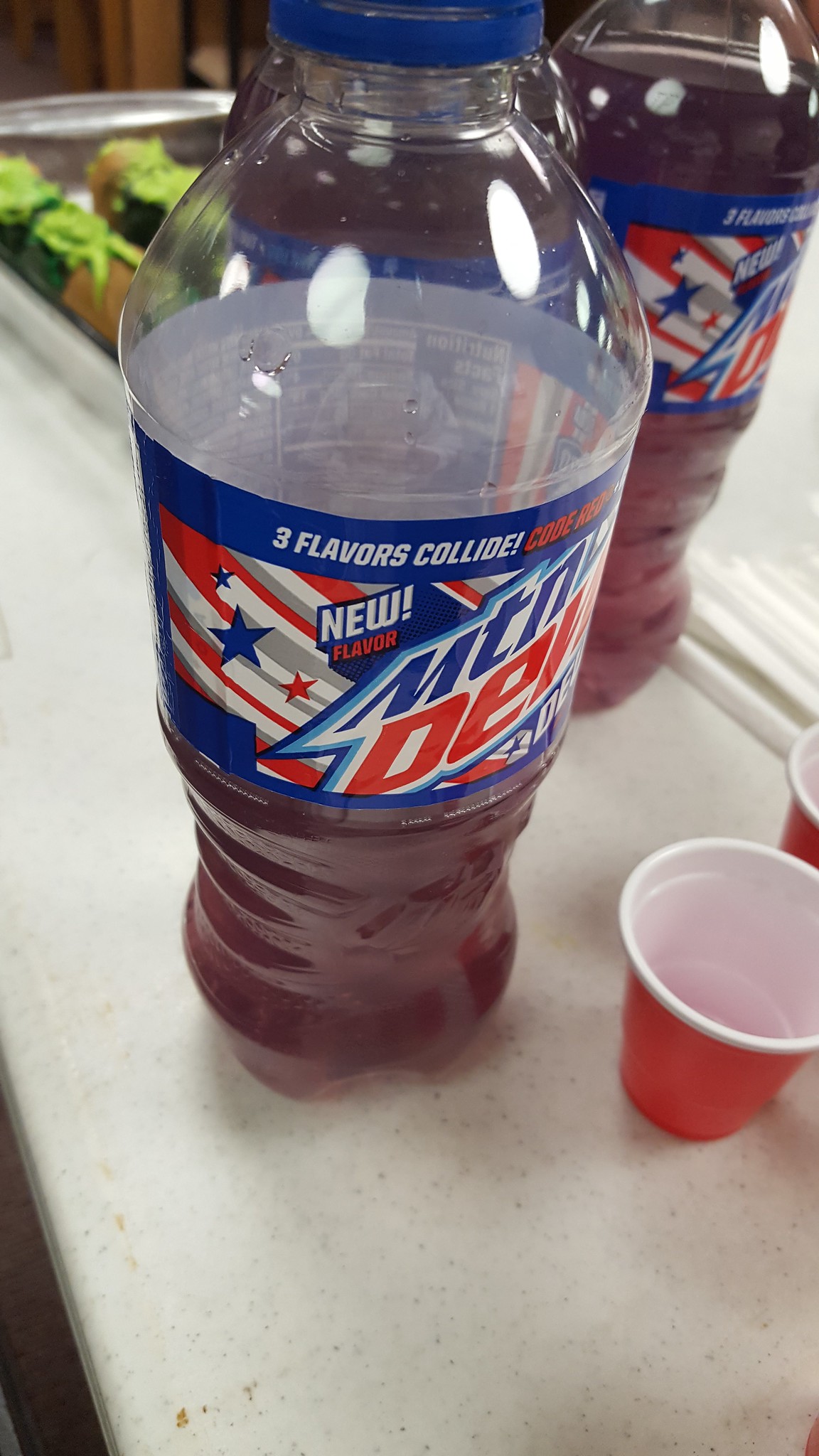In the image, a white countertop with black speckling serves as the base for an arrangement of items. Prominently displayed are two red cups, positioned to the right side of the image. On the left, a collection of brown pastries with a distinct green topping is visible. The focus of the image is on several drinks prominently featuring Mountain Dew's new flavor, "Code Red"—a vibrant red beverage. Text at the top of the image announces the new flavor release, highlighting a patriotic theme. The Mountain Dew logos incorporate blue and red colors, evoking the American flag, complete with white rectangles, blue stars, and red stripes, adding to the festive nature of the scene. Reflections of the drinks and cups are subtly visible on the glossy countertop, accentuating the vivid colors and festive feel.